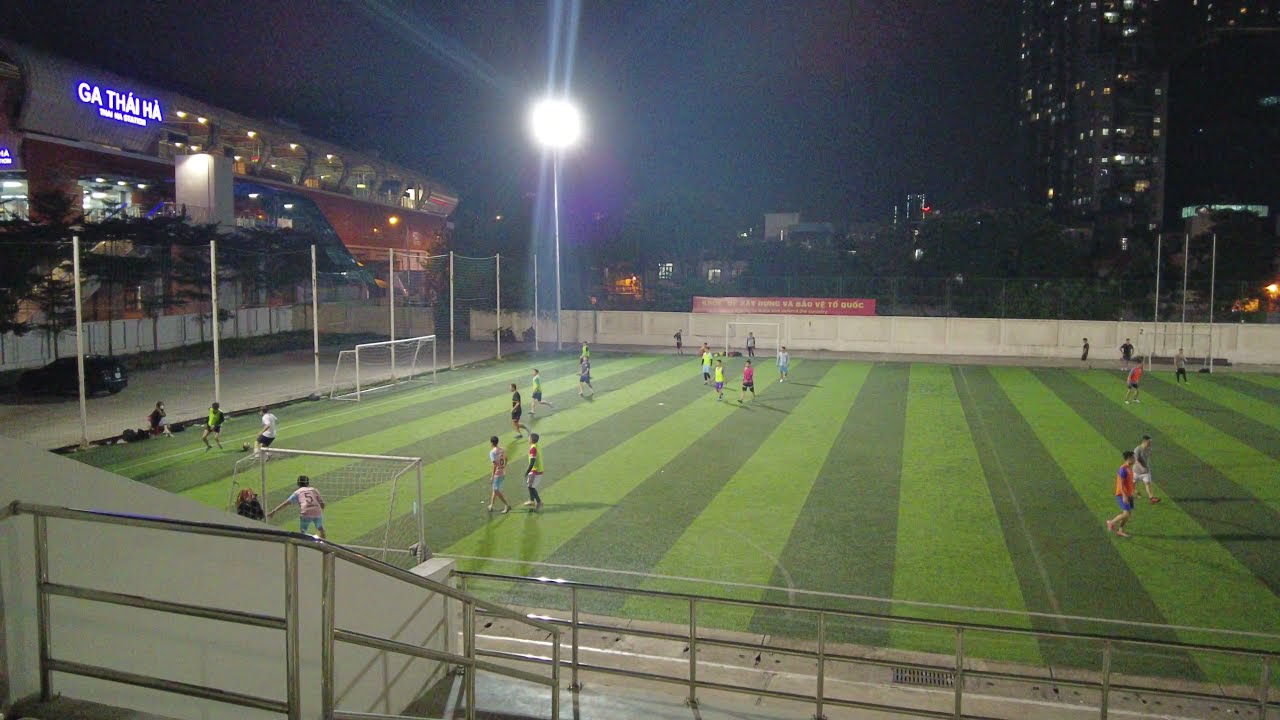This nighttime outdoor photograph captures a vibrant soccer field divided into light green and dark green vertical stripes. Multiple games are taking place simultaneously, with several nets positioned in different directions, indicating a practice session. The field is teeming with dozens of soccer players, all illuminated by a nearby street lamp in the center left, which casts a bright white light with a starburst effect. In the top portion of the image, the black sky frames the scene, while on the right, the lights of a towering skyscraper pierce through the darkness. To the left, a row of shops is visible, with a prominent blue sign that reads "Ga Thai Ha" in capital white letters, though the smaller text below is unclear. A shiny metal railing runs along the foreground, marking the elevated position from which the photo was taken. The scene also includes elements such as apartment buildings, stadium structures, a chain-link fence, and variously colored objects like blue, red, yellow, light blue, and pink, all contributing to the lively atmosphere of this urban soccer night.